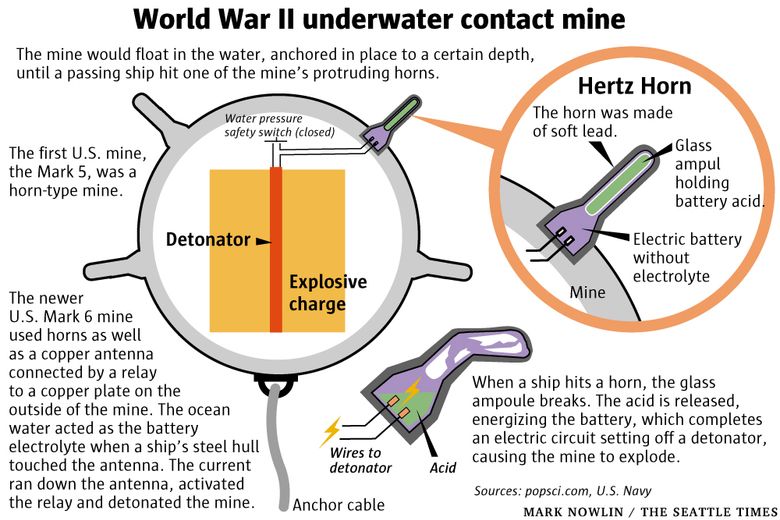This horizontal image, which lacks an external border, is an explanatory diagram on how a World War II underwater contact mine operates. At the top, in bold black print, it states, "World War II Underwater Contact Mine." The detailed captions below explain that the mine would float in the water, anchored at a specific depth, until a passing ship struck one of the mine's protruding horns. 

The image includes several diagrams and significant amounts of text. To the left, there is a depiction of the mine with protruding horns, illustrating its internal components: an explosive charge and a red-line-labeled detonator connected to each horn. A close-up of the horn details the wiring leading to the detonator.

Additionally, the image displays two highlighted sections: a left diagram encircled in gray showing the horn with a yellow background labeling the detonator and explosive charge, and a right diagram within a gold circle labeled "Hertz Horn." This section specifies that the horn was crafted from soft lead and contained a glass ampoule holding battery acid, an electric battery without electrolyte, and wires to the detonator. Beneath the illustrations, it further describes the mine's function and at the bottom credits Mark Nowlin from The Seattle Times.